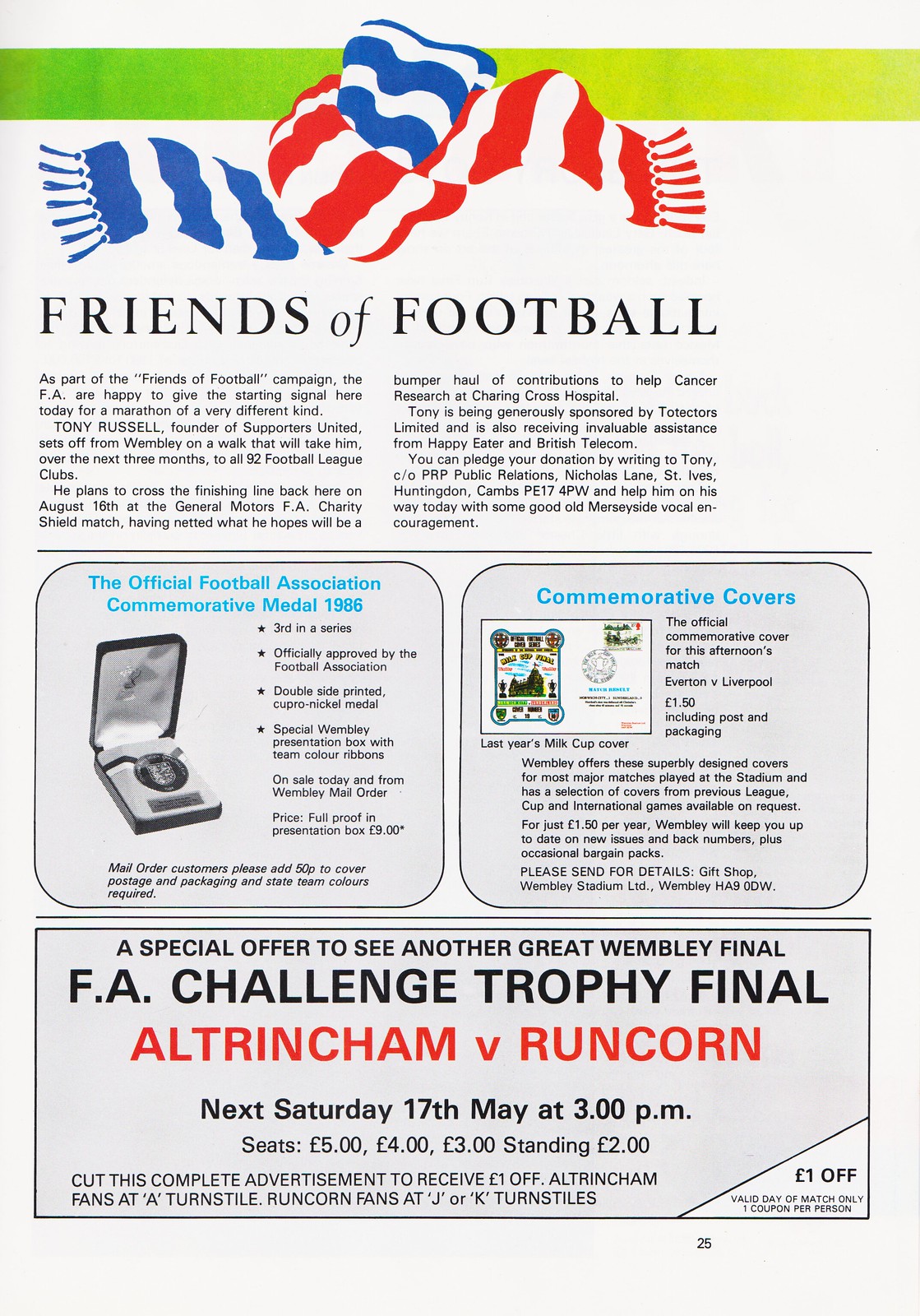The image is a color photograph of a promotional flyer for the Friends of Football campaign, printed on white paper with green, red, blue, and black ink. At the top, a green horizontal band runs across the flyer, below which are two intertwined scarves—one blue and white striped and the other red and white striped—knotted together. Beneath the scarves, in bold black letters, is the heading "Friends of Football." 

Following the heading, there are descriptive paragraphs that outline the Friends of Football campaign, mentioning its initiation by the Football Association (FA) and the campaign's purpose. Below these paragraphs, a thin black horizontal line separates the top section from three advertisements.

The upper left quadrant features the Official Football Association Commemorative Medal 1986, described as the third in a series and officially approved by the Football Association, with a black and white picture of the medal. The top right quadrant highlights Commemorative Covers with a small illustration. 

At the bottom of the flyer, another thin black horizontal line divides the advertisements from a larger box promoting a special offer. This section, outlined with a black border, advertises the FA Challenge Trophy Final, an upcoming football match between Altrincham and Runcorn, scheduled for Saturday, 17th May at 3 p.m. The promotion includes various ticket prices in pounds and details a coupon offering a one-dollar (or possibly one-pound) discount on match tickets.